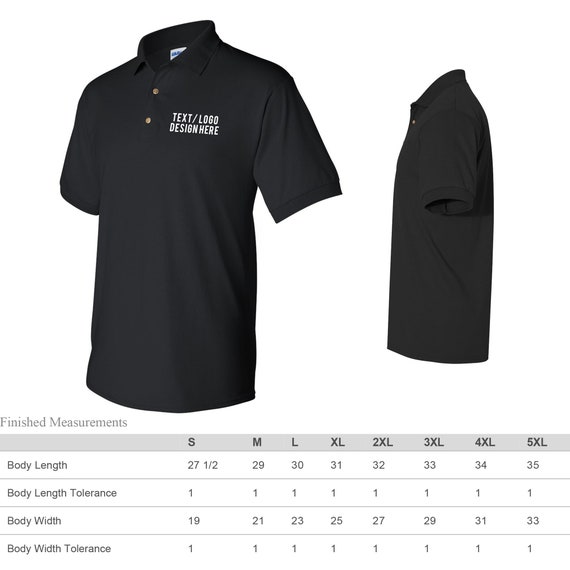This image, resembling a webpage with a white background, displays a detailed size chart for a dark blue, collared short-sleeved polo shirt featuring two buttons at the top. The shirt is depicted from both the front and side views. Notably, the front view features a white text/logo design located on the upper left chest area. Below the shirt images, a comprehensive size chart is presented, framed by a gray border at the top stating "finished measurements." The chart includes four key rows labeled body length, body length tolerance, body width, and body width tolerance, each with corresponding measurements for sizes from Small (S) to 5XL. Specifically, body length ranges from 27.5 to 35 inches, while body width spans from 19 to 33 inches. The tolerance for both body length and body width remains consistent at 1 inch across all sizes.